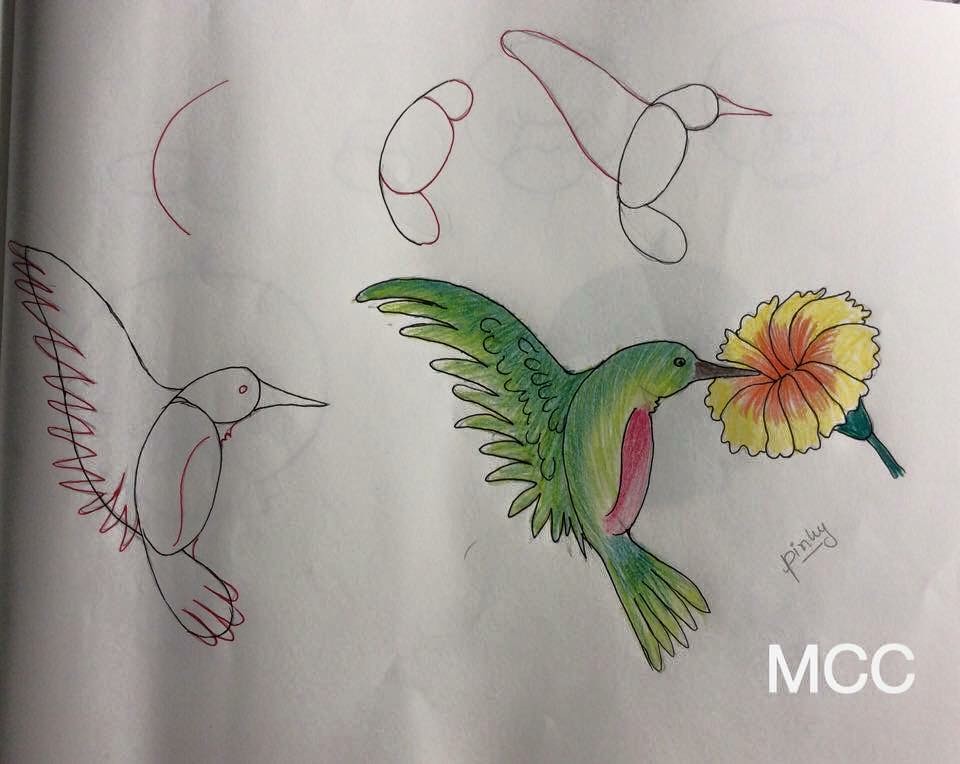The photograph depicts a detailed step-by-step drawing tutorial illustrating how to draw and color a bird. The progression starts from the upper left, with the initial drawing showcasing a simple line. Moving to the right, additional curves are added, gradually outlining the bird's body in sections. This continues to the next drawing where the wing shapes are incorporated. In the bottom sequence, further detailing is shown including the outlining of the bird's form in black and red ink.

The final drawing, situated towards the middle-right of the white paper, is a fully colored illustration of a hummingbird. The bird is depicted with a green body and a red breast, delicately feeding on a yellow flower with an orange center, which sits atop a green stem. The final artwork is signed "Pinky" with a small underline, positioned beneath the bird and the flower. Additionally, there's a watermark labeled "MCC" in white text at the bottom right corner of the page.